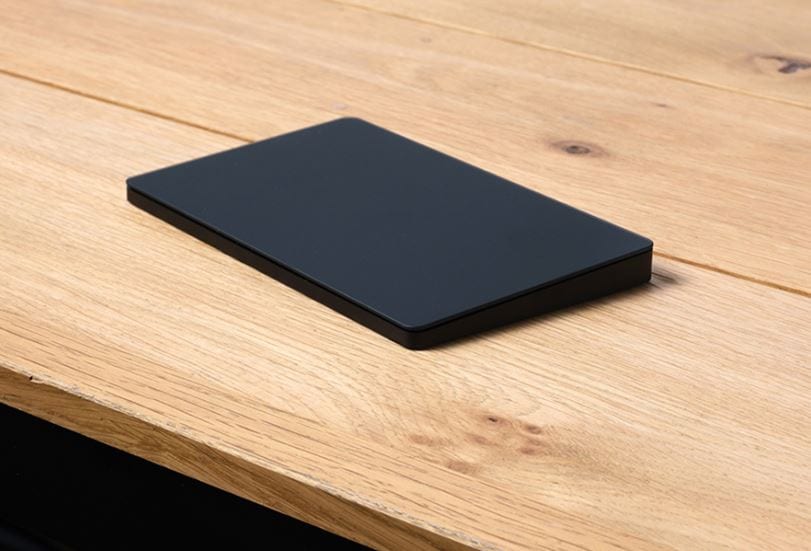The image showcases a light brown wooden desk composed of three distinct panels, resembling a picnic table structure. The wood grain patterns are visible, including darker circular knots adding a rustic charm to the surface. Positioned on the desk is a flat, rectangular black object, devoid of any text or logos, with a lid that suggests it could be an electronic device like a laptop or binder, though its exact nature is unclear. The desk sits on a black floor, and the overall lighting is flat, indicating that the photograph was likely taken indoors under fluorescent lights.